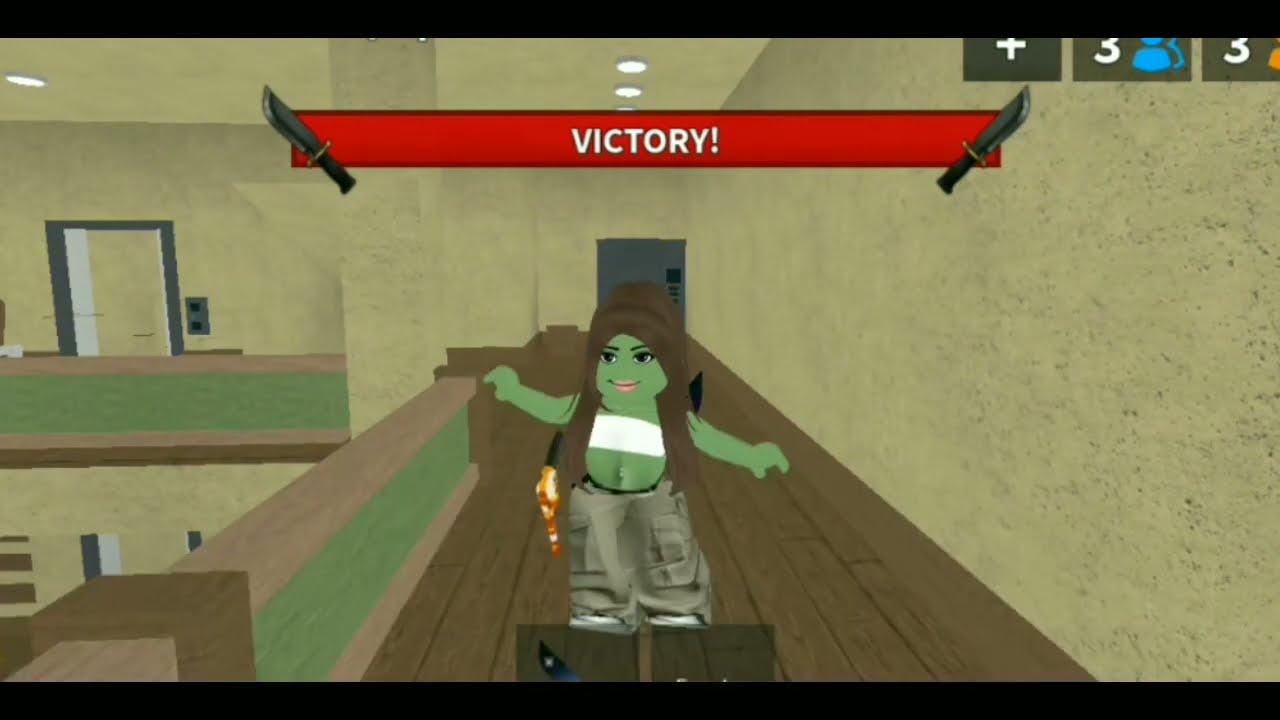The image is a detailed screenshot of a video game. Front and center stands a gremlin or frog-like female character with green skin, adorned in a white bandeau, oversized gray pants, and long brown hair. She appears to be equipped with a flamethrower on her back. The setting is an open-air second story of a building with sand-colored walls and hardwood flooring. From the character's position, a long hallway stretches behind her leading to a doorway, and to her left is a green and brown railing. Above her, a vibrant red banner displays the word "Victory," flanked by illustrations of knives. Additional items in the image include icons with the number three, one blue and one orange, near the banner. The scene, rich with colors like green, brown, tan, and gray, conveys the aesthetic of a low-budget video game.